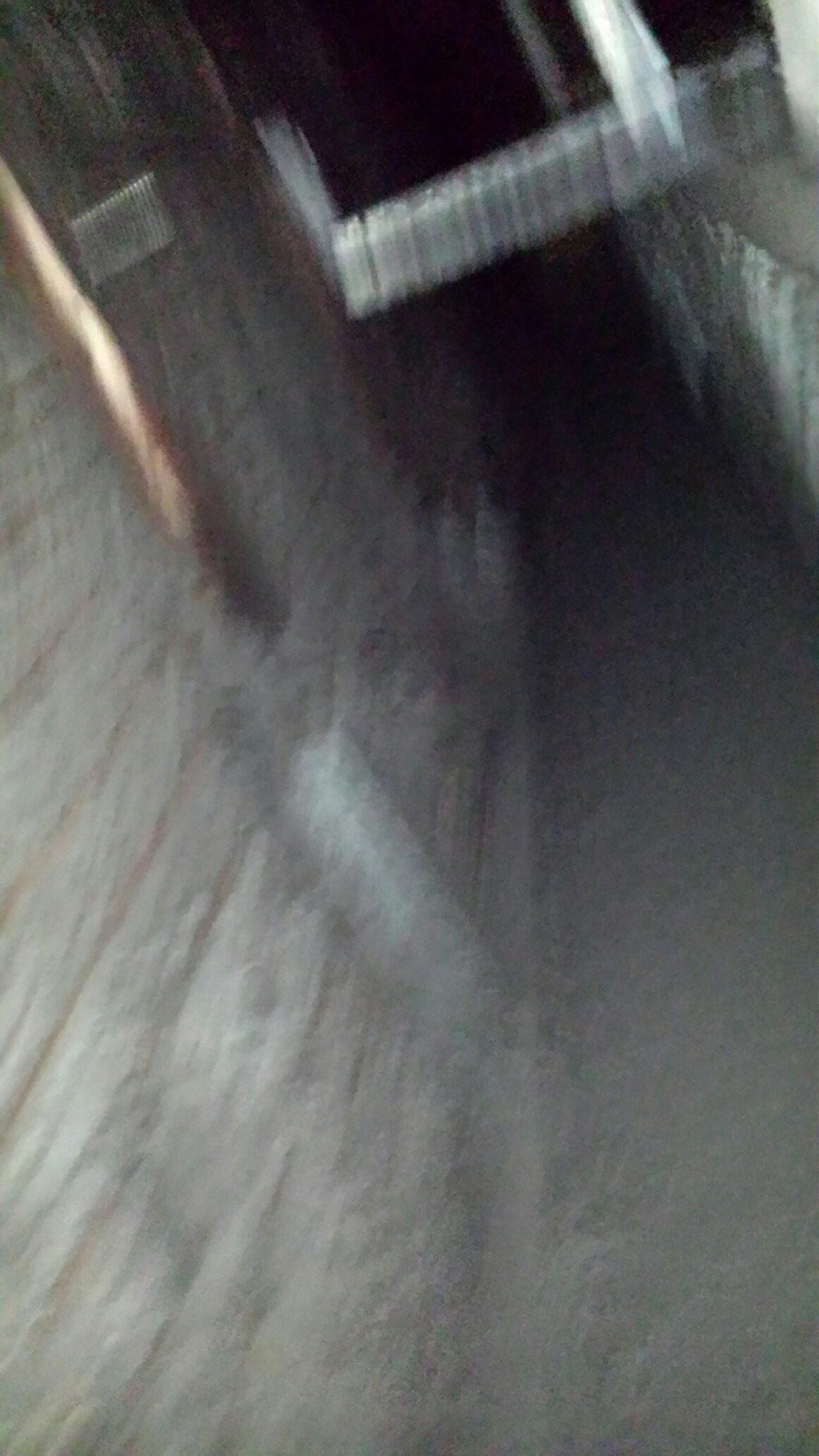In this image, a dimly lit and hazy street corner is depicted, characterized by its blurriness and vague details. On the left side of the image, a long, straight copper tubing, likely used for plumbing, runs along the side of a building or the street. Moving towards the horizon, the scene fades into pitch blackness. Just before this darkness, in the middle of the image, there is a noticeable divider or small bridge. This structure appears to be a thick iron beam jutting out from the top right of the image, extending all the way to the left where it meets the wall. The overall atmosphere is one of obscurity and dimness, making it difficult to discern finer details.